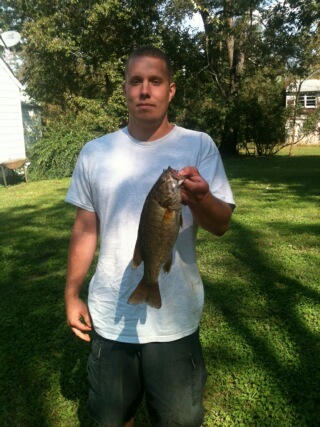In this outdoor photograph taken on a bright, sunny day, a man with a buzz cut and short blondish hair stands on a lush green lawn. He wears a white short-sleeve t-shirt and black cargo shorts or pants, which are cut off at the knees in the image. With a serious, neutral expression, he looks directly at the camera while holding a medium-sized, dark greenish-brown fish by its mouth in his left hand. His right hand rests near his pocket. Shadows from surrounding trees dapple the grass, suggesting a sunny day. In the background, to the top left of the image, the back of a white house with a possible satellite dish on top is visible. Further behind, there is a cluster of tall bushes and thick trees, and to the top right, another house with brown siding and a tiled roof can be seen in the distance.